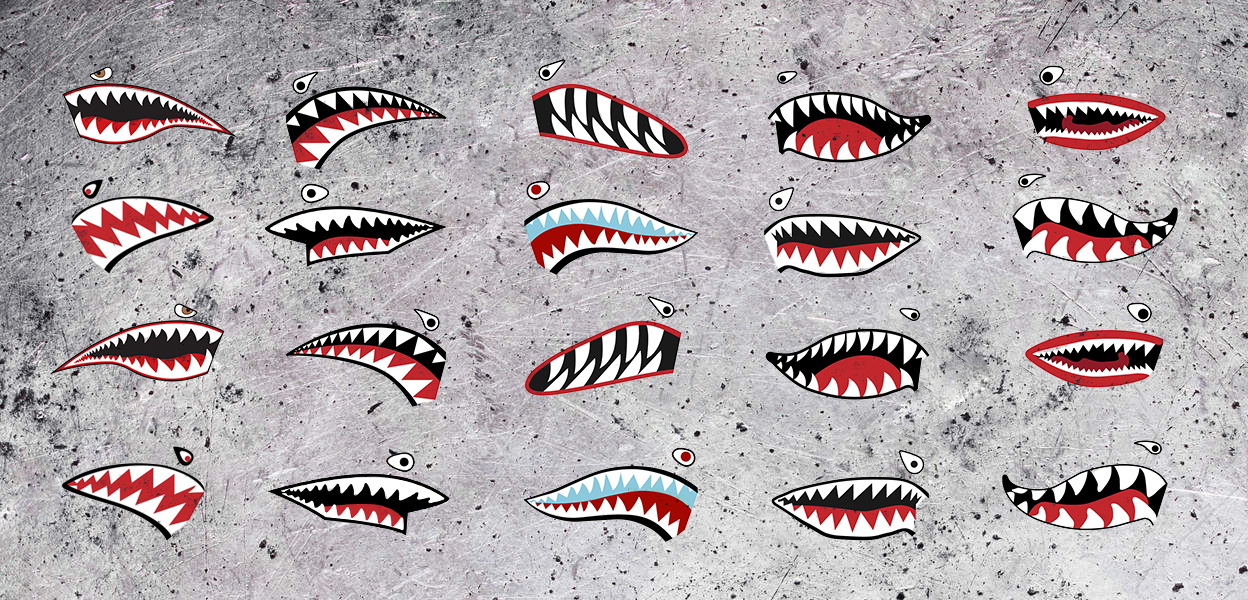The image depicts twenty different, monster-like mouths, each adorned with sharp, white teeth and a single eye. The mouths are set against a distressed, light gray concrete or metal-patterned background, possibly featuring graffiti art. The tongues in these mouths are predominantly red, and each mouth is drawn in a distinct, unique style. The mouths exhibit menacing expressions, further emphasized by their angry, bared teeth. The eyes are positioned variably: the top row features eyes on the left side, while the bottom row has them on the right. Most of the eyes are black and white, although some have red pupils and two in the center show a bit of light blue amidst the black within the mouths. These artistic decals or drawings collectively present an array of fearsome shark-like mouths.